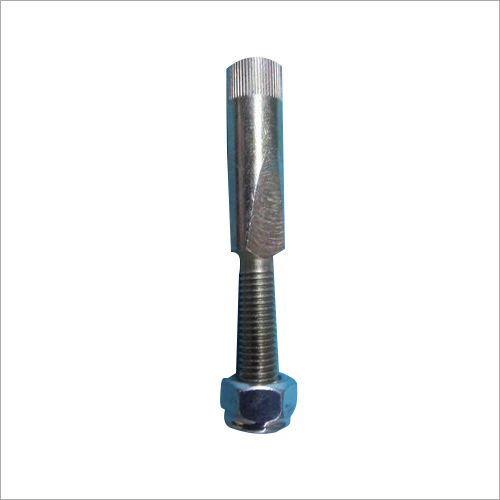The image showcases a highly detailed metal bolt and nut assembly, presented against a plain white background. The bolt has a shiny, gray-silver metallic finish and features a threaded cylindrical shaft that extends upwards. At the base of the bolt is a nut with a distinct blue hue, possibly due to bluish tape or paint, adding a touch of color to the predominantly gray composition. This nut has a rounded and beveled design and extends slightly at the bottom. Both the bolt and nut appear to be made of metal, reflecting light to give a clean, polished look. The bolt's upper end is detailed with a vertically striated grip pattern, providing textural contrast and functionality for easy handling. The entire object stands out crisply against the stark, unbroken white background, making it a clear and vivid representation of the metallic assembly.